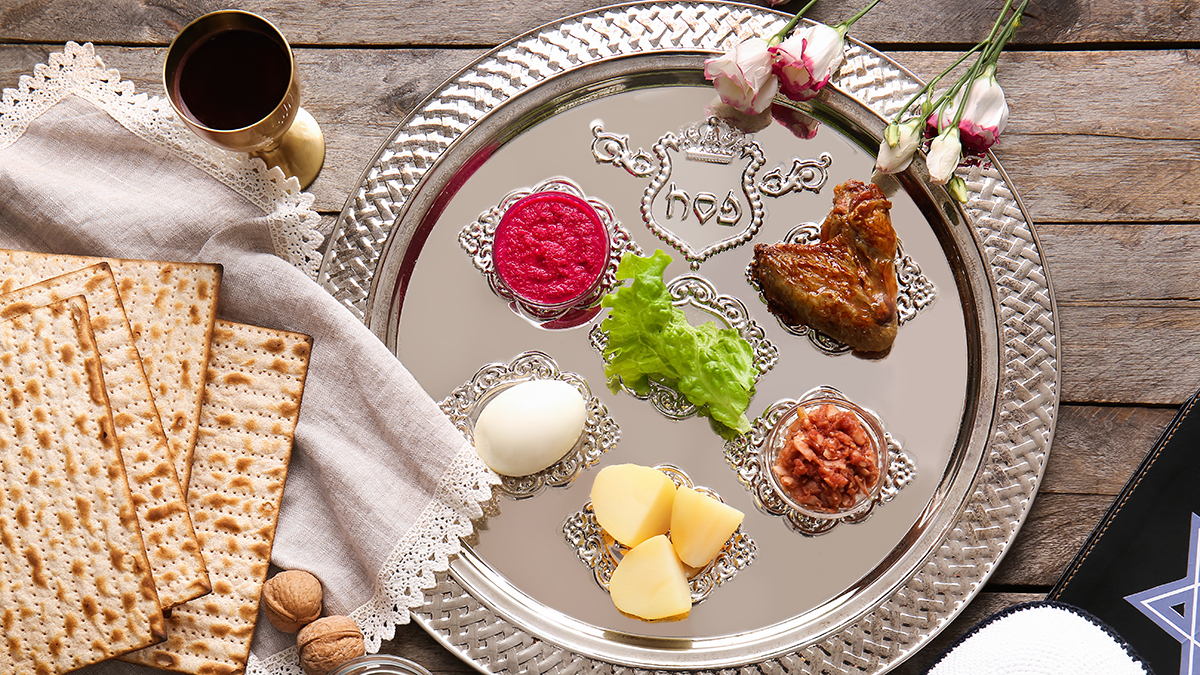This top-down photograph, possibly AI-generated due to its slightly unrealistic appearance, depicts a rustic wooden table with a light brown-grayish tone. At the center of the image is an ornate silver plate featuring raised, beaded designs that demarcate sections for various foods. Among these sections, we see traditional Jewish festival items: a piece of chicken, an egg, lettuce, three pieces of potato, a red dipping sauce, and possibly fried onions. Surrounding the edge of the plate are five white roses with red tips, adding a decorative touch. To the left, on a beige lace napkin, rest four pieces of matzah and a couple of walnuts, accompanied by a small, reflective gold goblet. On the right side of the image, there is part of a cloth bearing a Jewish symbol, anchoring the festival ambiance communicated through the various items displayed.